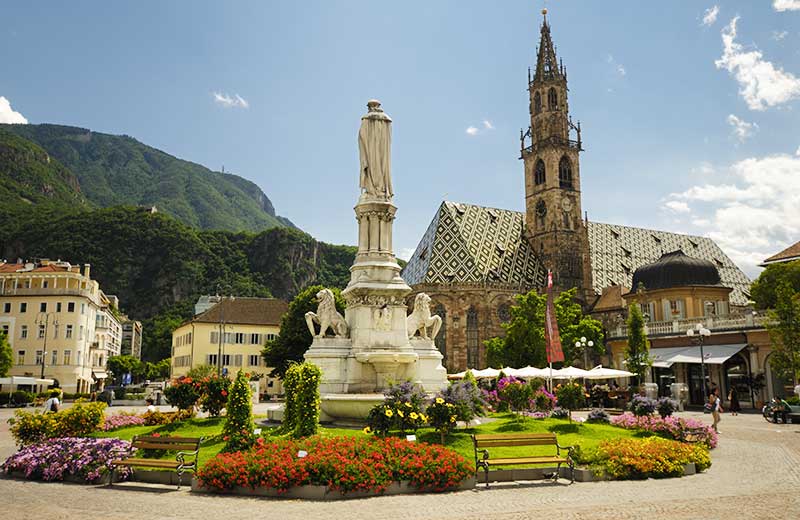The image depicts a picturesque outdoor area blending nature, architecture, and vibrant town life. In the foreground, there is a traffic circle that doubles as a lush garden. This central area is beautifully landscaped with a variety of colorful flowers and bushes, encircled by grassy patches and wooden benches. Dominating the scene is a magnificent white statue featuring a robed figure standing atop, flanked by lions at its base.

Surrounding this serene garden, the town’s skyline is framed with diverse buildings. Prominently, an ornate, old church with a towering steeple hints at its historical significance, while its intricate roof design adds to the town's charm. Adjacent to the church, an outdoor cafe with umbrellas and an awning suggests a cozy spot for visitors, though tables are obscured by the lush plant life.

Further back, several multi-storied buildings, some of them yellow, blend harmoniously into the verdant, tree-covered mountains that form a scenic backdrop. The left side of the image features a rugged, forested hillside, adding to the natural beauty of the area. The sky overhead is mostly clear, showcasing a deep blue expanse with a few fluffy clouds drifting by. Several people are seen strolling along pathways to the right, enhancing the lively yet tranquil atmosphere of this charming European-like town.